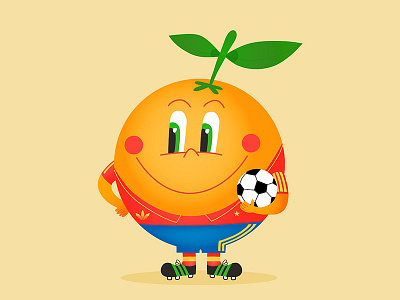In this cartoon-style illustration, we see an anthropomorphic orange standing at the center of the image against a flat cream yellow background. The orange character is spherical in shape and sports a stem with two leaves protruding from the top of his head, one pointing in each direction. He has a charming face with arched, oval-shaped eyes—rounded at the top and flat at the bottom—featuring green irises and black pupils. His thin, orange eyebrows and a smiling, thin reddish-orange mouth enhance his cheerful expression, complemented by red dimples on either side of his large smile. His nose is also a small, arch-shaped, reddish-orange feature.

The orange is dressed in a sporty red shirt with yellow accents and an Adidas logo, indicating it's a soccer shirt. He pairs this with blue shorts that also have yellow accents. His red and yellow socks match the overall color scheme, and he completes his outfit with black and green cleats. In his rightmost arm, he holds a black and white soccer ball, reinforcing the sporty theme. This vibrant and detailed portrayal of the orange character emphasizes his joyful and athletic nature.